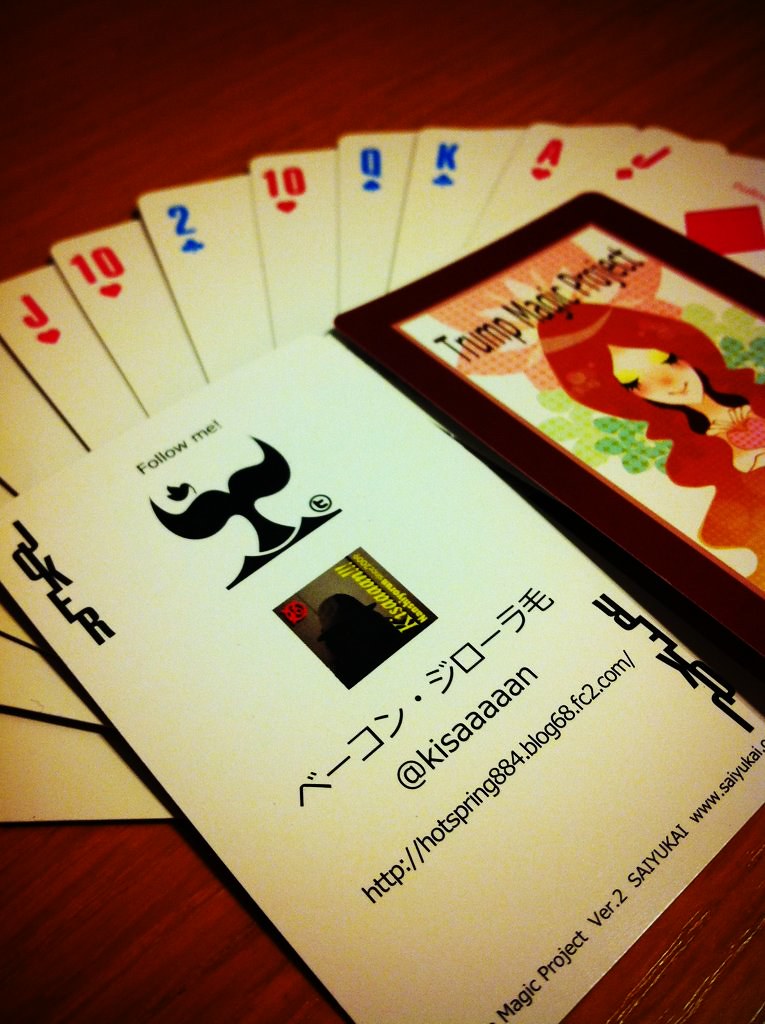The photograph showcases a deck of playing cards elegantly arranged on a light-colored wooden surface, allowing the distinct wood grain to be clearly visible. The cards are fanned out at the top of the image, displaying a variety of suits and colors. Notably, this particular deck features blue clubs instead of the traditional black, distinguishing it from conventional playing cards. Among the visible cards, we can identify a jack of hearts, ten of hearts, two of clubs, queen of spades, king of clubs, ace of hearts, and jack of diamonds.

Prominently positioned atop the fanned-out cards is a joker card, which includes an advertisement with the URL "hotspring884.blog68.fc2.com" and the phrase "follow me," suggesting it may be related to the manufacturer or a promotional campaign. Additionally, there is another distinct card that appears to showcase the reverse side of the deck, adorned with an animated image of a female figure with long hair, alongside the text "Trump Magic Project." This indicates the thematic design present on the back of the cards, adding an artistic and enigmatic touch to the deck.